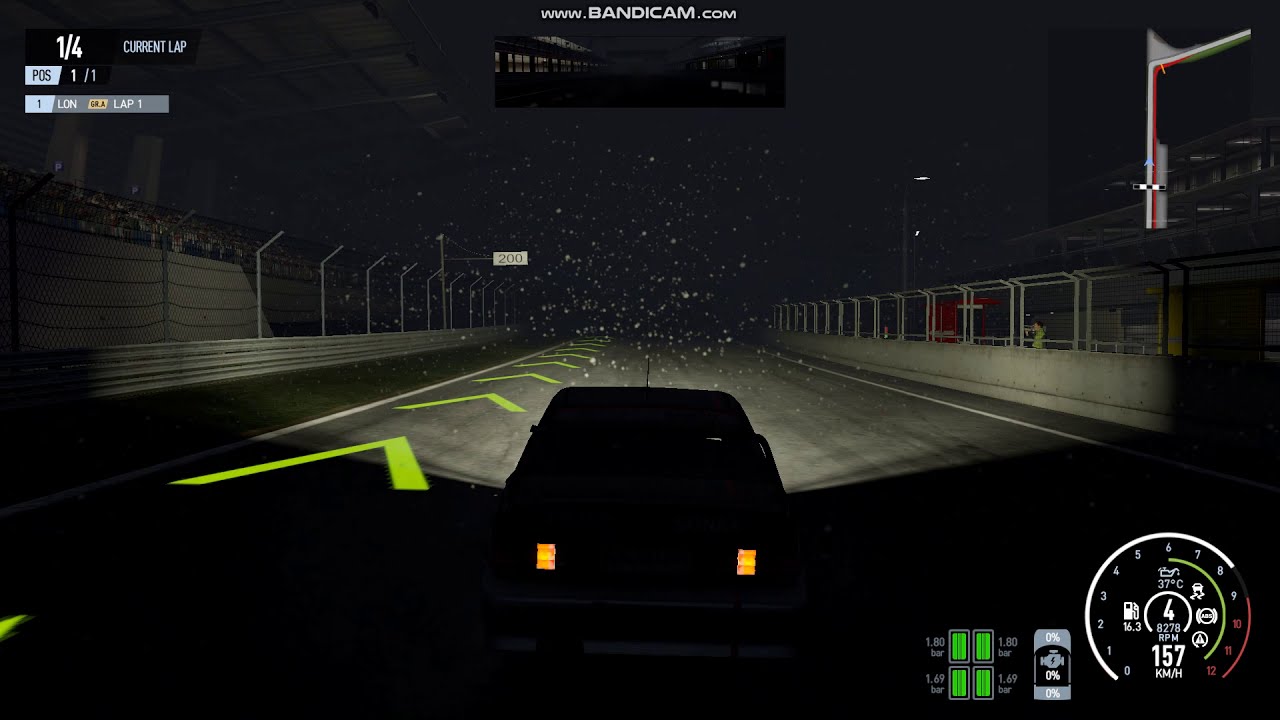The image depicts a nighttime scene from a racing video game, captured from a third-person perspective. Central to the image is a car visible from the back, with its silhouette discernible and brake lights glowing orange. The car is speeding down an empty, snow-covered road flanked by fencing and guardrails—metal on the left and concrete on the right. Left of the car, yellow directional arrows can be seen receding into the distance, and a white sign with "200" is faintly visible. There are also indistinct stands filled with people to the left. The only light in the immediate vicinity comes from the car's headlights illuminating the path ahead, although distant streetlights are also visible. The bottom right corner of the image displays a detailed heads-up display (HUD) with a speedometer showing the car traveling at 157 kilometers per hour, oil and gas gauges, ABS lights, and a reading of 8278 RPMs. The top left corner shows a fraction "1/4," and the top edge features a website URL, "www.bandicam.com." The road appears to be a bridge, considering the fencing on both sides, heightening the immersive racing experience in the snowy night setting.